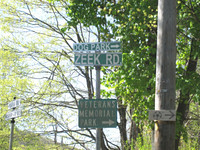In this small, outdoor photograph taken during daylight, a prominent signpost adorned with various directional signs captures the viewer's attention. The most noticeable sign, in green with white trim and white letters, reads "Zeke Road." Above it, a smaller but similar green sign with white trim and lettering indicates "King Park." Adjacent to the signpost, a parallel wooden pole with a smooth surface is visible, to which a loosely attached sign featuring an arrow pointing in one direction is affixed. The background reveals a mixture of trees, some vibrant with green leaves, while others are nearly bare. The sky is overcast, presenting a white, cloudy appearance that further emphasizes the outdoor setting.